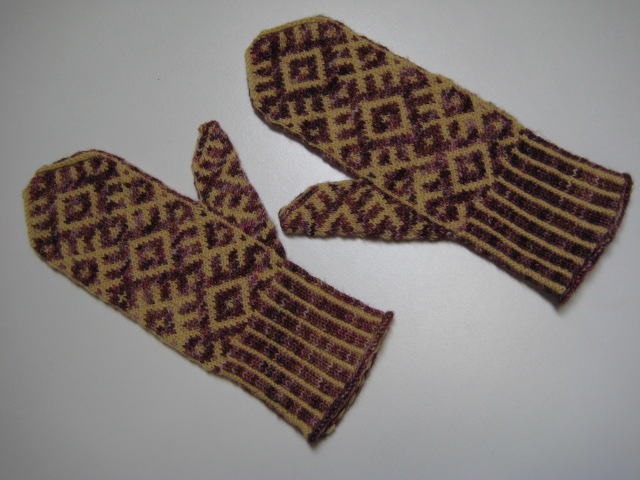The image showcases a landscape-oriented color photograph of a pair of intricately knit mittens, laid at an angle from the top left to the bottom right, with their thumbs pointing towards each other. These mittens exhibit a traditional Scandinavian design, potentially Selbu-style from Norway. The primary color is a light gold or cream, contrasted with variegated hues of purplish, pinkish, brownish, and reddish tones. The top of the mittens features a detailed diamond pattern that continues onto the thumb, with smaller diamonds nested within. The cuffs are deep and adorned with alternating stripes in a textured pattern of three knit stitches in the colorful variegated yarn to one purl stitch in cream. The cuffs also display a contrasting weave of dark brown with light gold striping. The mittens are displayed on a gradient gray background, enhancing the colors and intricate details of the knitting. The style of the photograph is a blend of photographic representationalism and realism, typical of high-quality product photography.